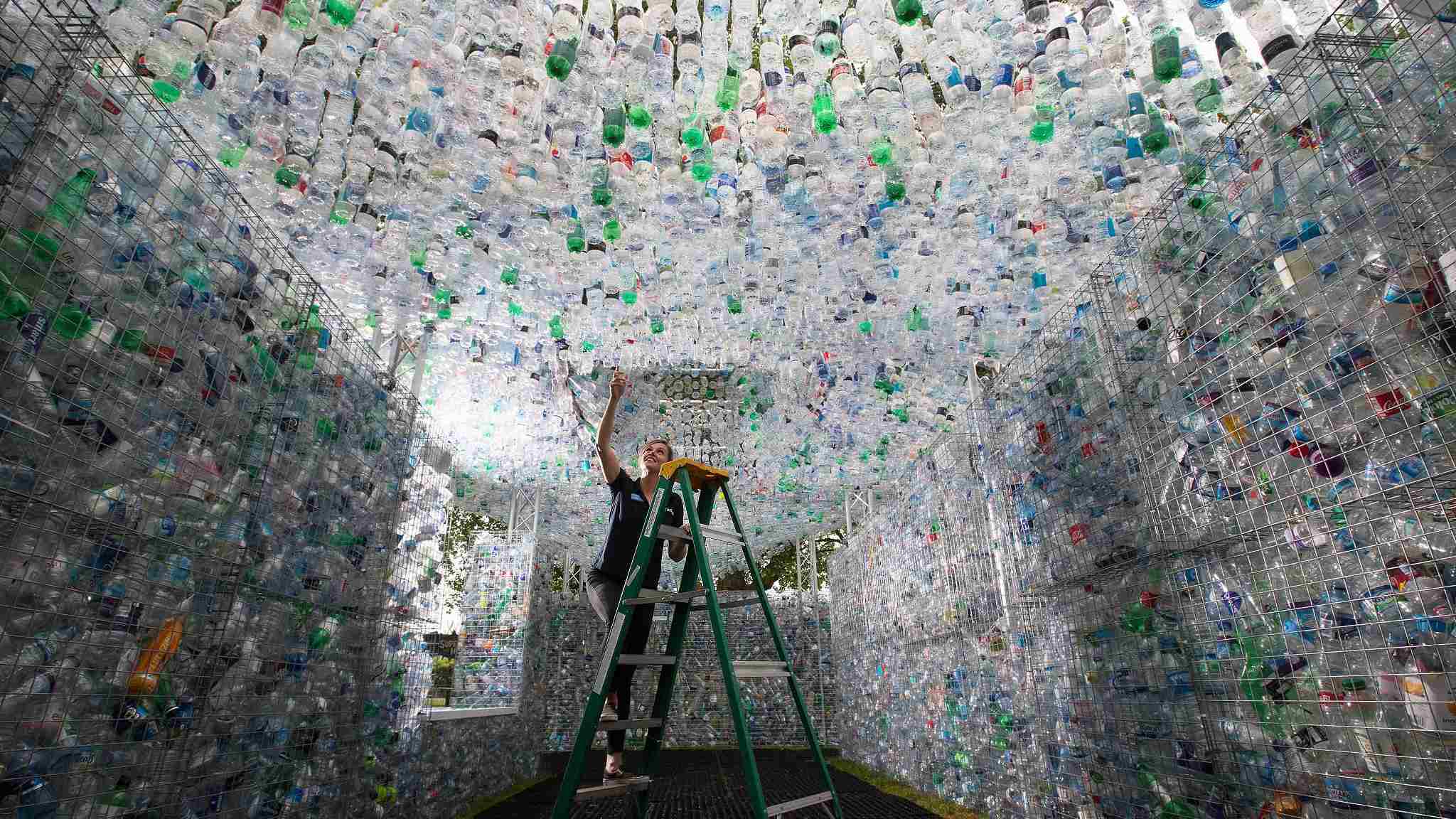In this image, we see a woman standing on a green step ladder in the middle of a room, engaged in a creative project. She is dressed in black clothing and sneakers, with her hands reaching up to touch a plastic bottle that is attached to the ceiling. The ceiling and walls of the room are covered with an intricate installation of plastic bottles suspended between metal wires. These bottles vary in type, including water bottles and green bottles resembling beer bottles. The overall impression of the room is a mix of sparkling and shiny elements, with some sections exhibiting silver, red, blue, and yellow hues, evoking the appearance of reflective tiles. The woman appears to be smiling, contributing to the sense that she is enjoying her artistic endeavor.